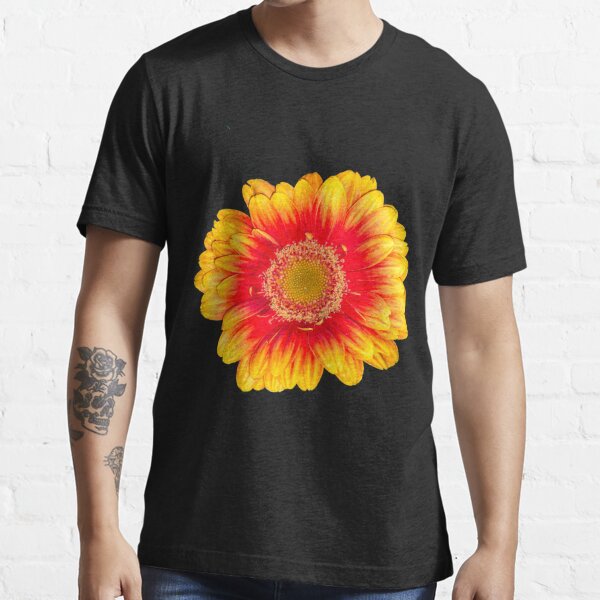The photograph features a close-up of a man standing in front of a white brick wall. The man is dressed in a black short-sleeved t-shirt that prominently displays a large and vibrant sunflower print. The sunflower is detailed with yellow outer petals, a ring of red towards the center, followed by an interior filled with green dots representing the seeds. The man is also wearing dark blue jeans, visible at the bottom of the image. His left arm showcases a tattoo of a rose emerging from a skull, while his right arm bears a tattoo of a roaring jaguar's head along with another partially obscured tattoo. The image captures the man from the neck down, revealing only the bottom of his chin. The bright colors of the sunflower on the t-shirt, contrasted against the white brick background, create a striking visual effect.